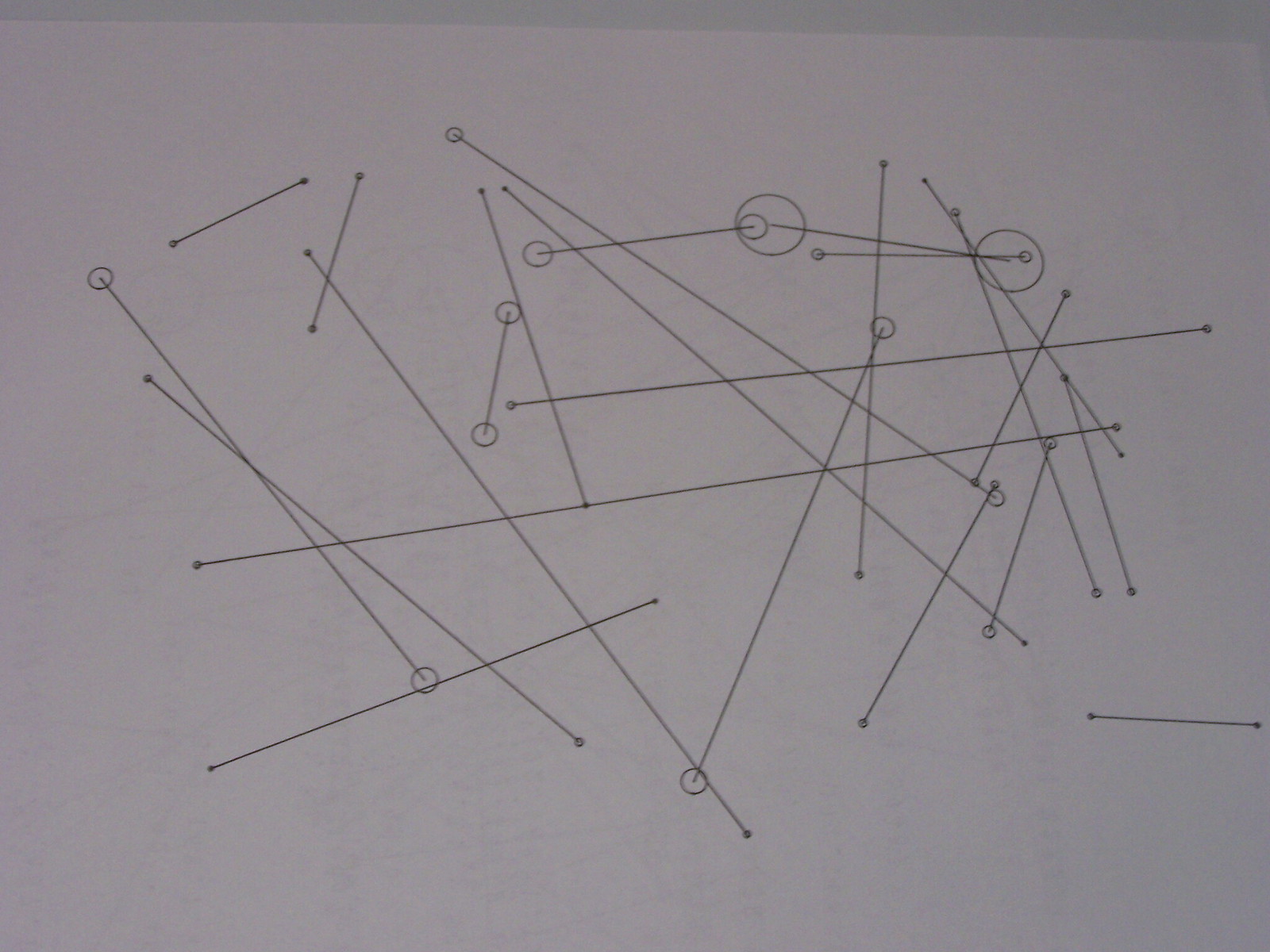This image captures a piece of standard computer paper with a series of meticulously sketched lines, set against natural lighting that gives the photograph a slightly dim appearance due to the absence of artificial light. Each line is perfectly drawn, and most terminate in a small circle or dot, with variations in the size of these endpoints. 

The lines appear overlaid in a manner similar to a scattered pile of needles or pick-up sticks, where each line partially covers another, yet remains distinctly visible. Notably, some lines feature larger endpoints, creating a striking contrast against those with tinier terminations. A particularly prominent line in the top-right quadrant boasts significantly larger circles at its ends, making it stand out among the rest.

In terms of distribution, the two smallest lines occupy the top-left and bottom-right quadrants. The lines intersect and crisscross in various directions, with one line forming a T-shape, running diagonally across the page. In the left third of the image, another line bisects this T-shaped line, also ending in a tiny circular point. The composition of intersecting lines, coupled with the variation in endpoint sizes, creates a complex and visually intriguing pattern.